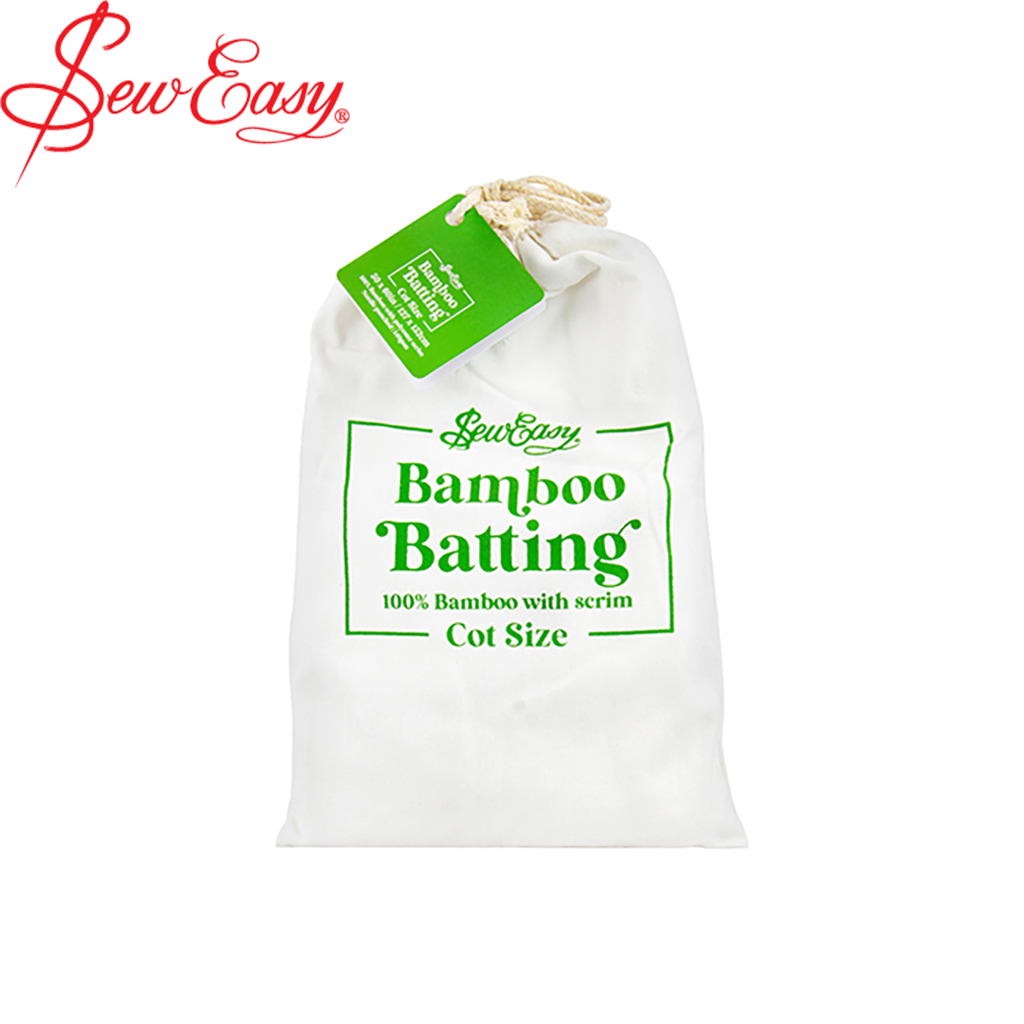The image showcases an advertisement for a product featuring a white, rectangular drawstring bag with a white rope closure. The upper left-hand corner of the image prominently displays the logo "Sew Easy" in red cursive text, with a needle threading through the 'S'. The same logo, in green text, is also displayed on the front of the bag. Below the logo, the bag's front text reads, "Bamboo Batting, 100% Bamboo with Scrim, Cot Size." A green tag attached to the top of the bag further reiterates "Bamboo Batting," although additional text on the tag is too small to read. Overall, the detailed focal point of the image is a neatly packaged white bag with distinct branding and product information, indicating it contains bamboo batting.